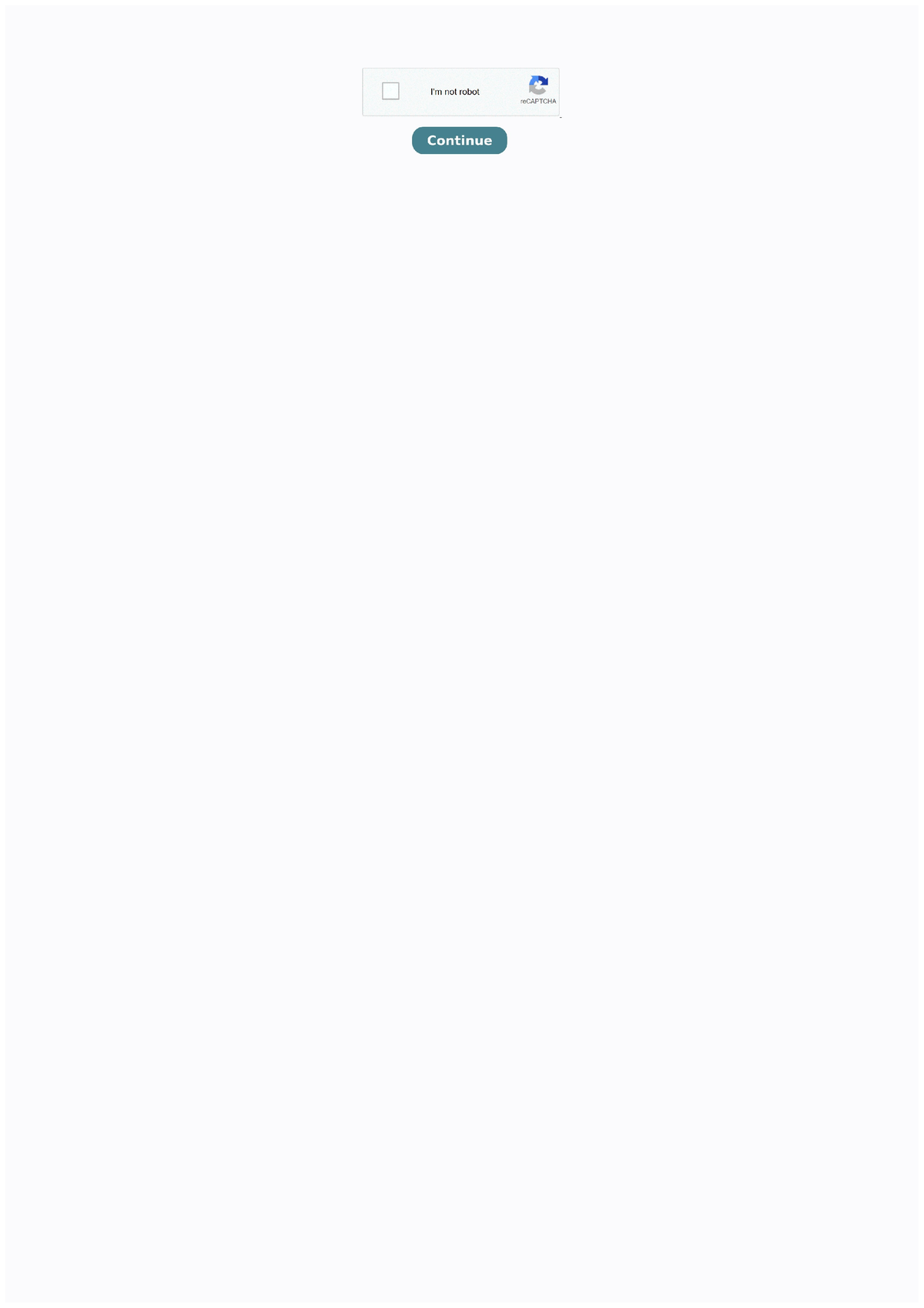The image depicts a minimalistic webpage with a predominantly white background. Centrally positioned near the top, there is a light gray rectangular box bordered in a darker shade of gray. To the right within this box, there is a square outlined in gray and featuring a white interior. Adjacent to the square, bold, dark text reads, "I'm not a robot."

On the far right side of the rectangular box, there is a circular icon with an arrow emerging from one end, accompanied by the text "ReCAPTCHA" underneath it. Below the rectangular box is another prominent element: a medium to dark blue rectangular button. This button features the word "CONTINUE" in white text centered on it.

The remainder of the page is blank, offering no additional symbols, images, or text, ensuring that the viewer's focus remains on the described elements.